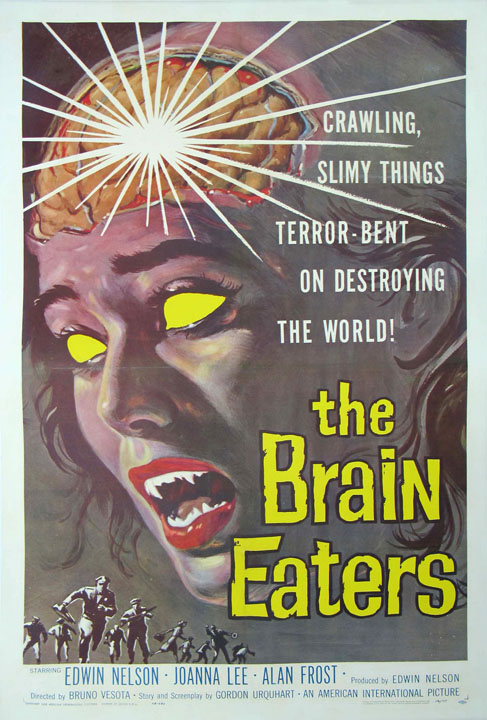**Detailed Caption:**

This image features a vintage movie poster for a film titled "The Brain Eaters." The poster is designed in a vertical rectangular format. The background gradients from a blackish hue at the top to a gray tone towards the bottom. Dominating the foreground is the side profile of a woman's head, primarily showing her left side with a slight front view. Her skin appears pale gray with a textured or swirled effect, and the top and back portions of her head are abnormally large.

The skull at the front of her forehead and the top is exposed, revealing her brain beneath. Bright white light emanates from her exposed brain, with rays extending outward. The woman’s dark hair is absent from the exposed areas, further emphasizing the eerie brain illumination. Her facial features include very dark eyebrows and glowing yellow eyes devoid of pupils, enhancing the sinister appearance. Her lips are painted a striking red, revealing very white, jagged, and sharp teeth, with especially elongated canines.

Occupying the bottom part of the poster, there are small figures of people running, indicating a sense of urgency and terror. The border of the poster is a light bluish-gray color. At the bottom, the names Edwin Nelson, Joanna Lee, and Alan Frost are prominently displayed, likely denoting the principal actors of the film. The woman's macabre visage takes up the majority of the poster, creating a haunting and unforgettable image reminiscent of classic horror movie artwork.